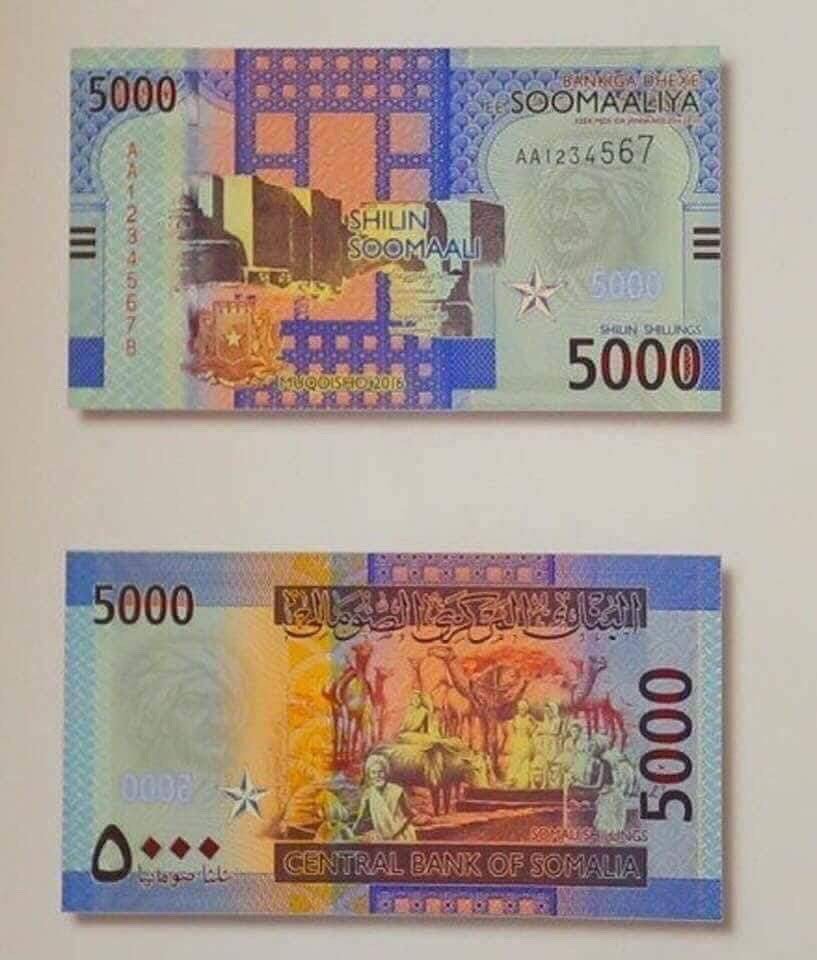The image showcases both the front and back of a 5,000 shillings note from Somalia. The front of the bill prominently displays the number "5000" in both the top right and bottom left corners and is labeled "Shillings" and "Somalia." Central imagery features a picture of a town, with additional elements such as a crest, a historical figure, buildings, and flags. The bill exhibits a blue and green color scheme, accented with orange, yellow, and white highlights. Arabic writing appears on the front and across the design. The back of the bill continues the blue theme and features intricate drawings, including people, camels, and possibly symbolic scenes. The words "Central Bank of Somalia" are clearly marked, along with additional foreign text. Both sides of the note are detailed and colorful, with red letters and numbers adding to the complexity of the design.